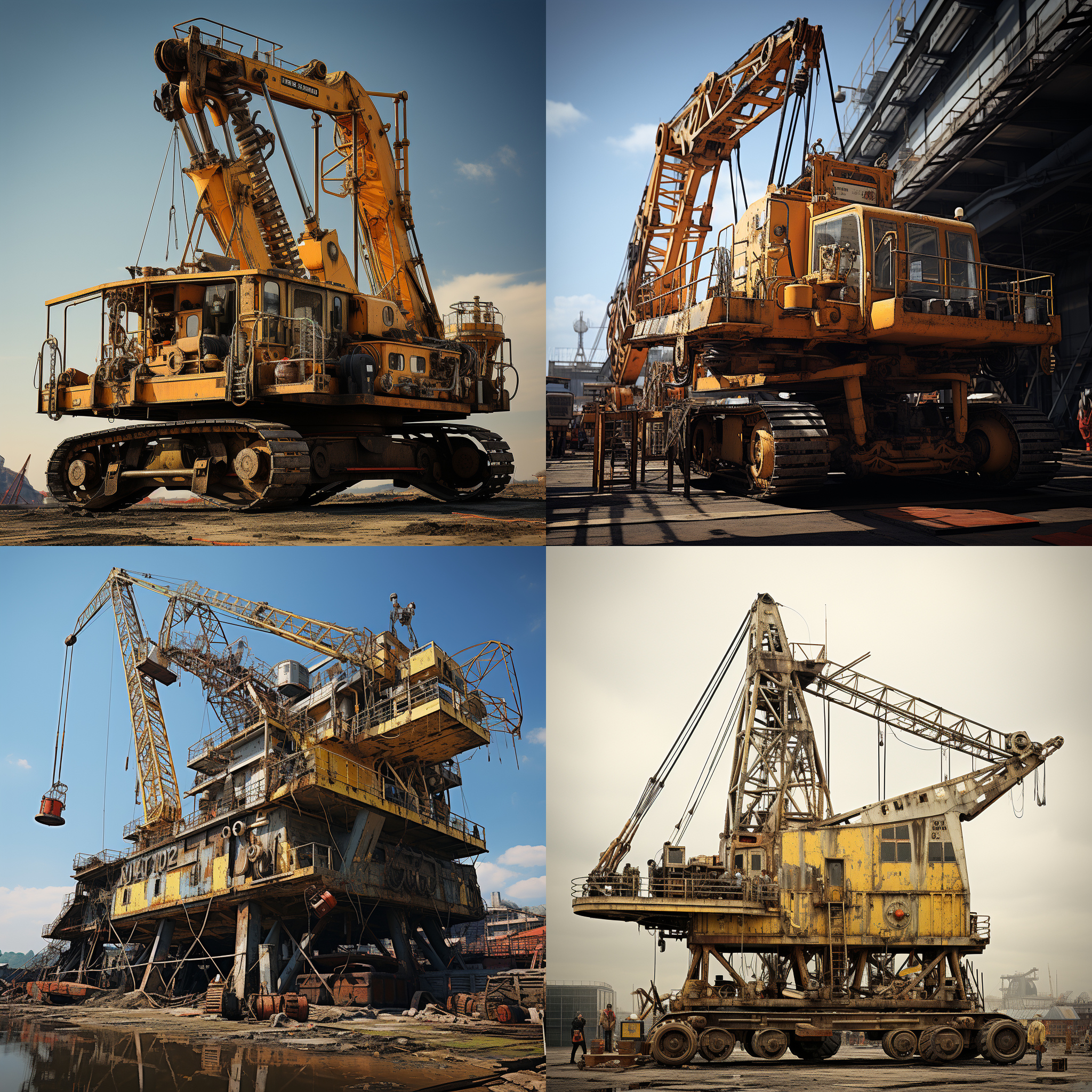The composite image showcases four separate photos of extensive, yellow industrial cranes, each occupying a quadrant of the square format. These towering cranes, which resemble the size and height of buildings, appear purpose-built for heavy-duty tasks such as bridge construction. All the cranes are equipped with extensive cabling systems and operator cabins, highlighting their complex machinery. The cranes are mounted on tracks instead of wheels, indicative of their capability to handle rugged terrains. Three of the images (top left, bottom left, bottom right) display visibly dirty and heavily used cranes, suggesting they are actively employed on dusty construction sites. In contrast, the top right crane appears cleaner, possibly indicating it is currently idle or recently maintained. In the bottom right image, human figures are seen adjacent to the machinery, providing a sense of scale and emphasizing their enormous size. Each snapshot is taken under daylight in an industrial or manufacturing setting, further detailing the cranes’ robust presence and operational state.